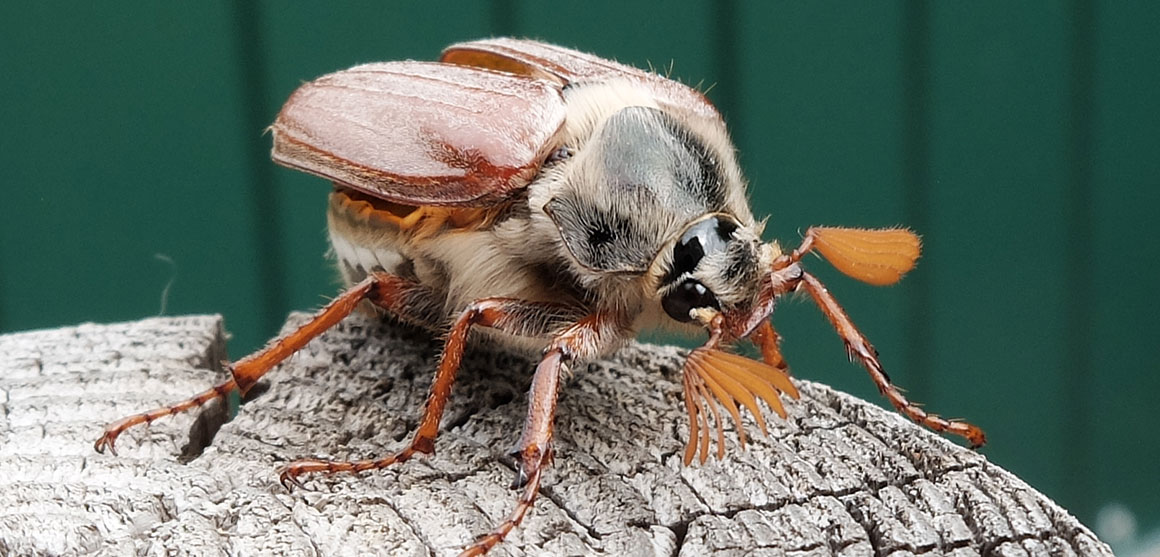This outdoor daytime photograph, approximately five inches wide and two to three inches high, captures a close-up of a beetle (possibly a maybug) perched on the top of an aged, flat-cut, rounded log. The background features a green, vertically slatted wooden fence or structure. The beetle is facing right, and its body exhibits fascinating details: a small black head with two black eyes and unique antennae extending outward, each with 6 or 7 light orange perpendicular extensions. The neck of the beetle is adorned with white fur that transitions into its back, where there are white and gray furry segments. Covering the beetle's back are two large, segmented, hard-backed brown wings with shell-like coverings. Its amber-colored legs, detailed with tiny white furs, extend out to the sides and down. The overall combination of colors—orange, tan, black, green, light brown, and beige—contrasts richly against the green background, making the beetle the undeniable focal point of this detailed and vibrant image.